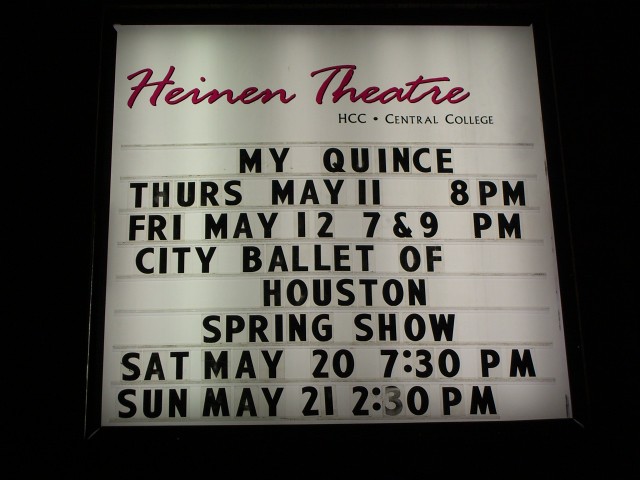This is a nighttime image of a theater marquee that is illuminated from within. The sign is predominantly white with a backlight, making the text clearly readable even in the dark surroundings. The top of the sign displays a permanent logo in red cursive that spells "Heinen Theater" (H-E-I-N-E-N T-H-E-A-T-R-E). Below the logo, in smaller black uppercase letters, it reads "HCC • CENTRAL COLLEGE." The sign advertises several events in all black slide-in letters: "My Quince - Thursday, May 11th at 8 p.m.; Friday, May 12th at 7 p.m. and 9 p.m.; City Ballet of Houston Spring Show - Saturday, May 20th at 7:30 p.m.; Sunday, May 21st at 2:30 p.m." The background is consistently white and lit up, with the light emphasizing the text and making it stand out starkly against the dark night. Horizontal gray lines also separate each event listed on the marquee.